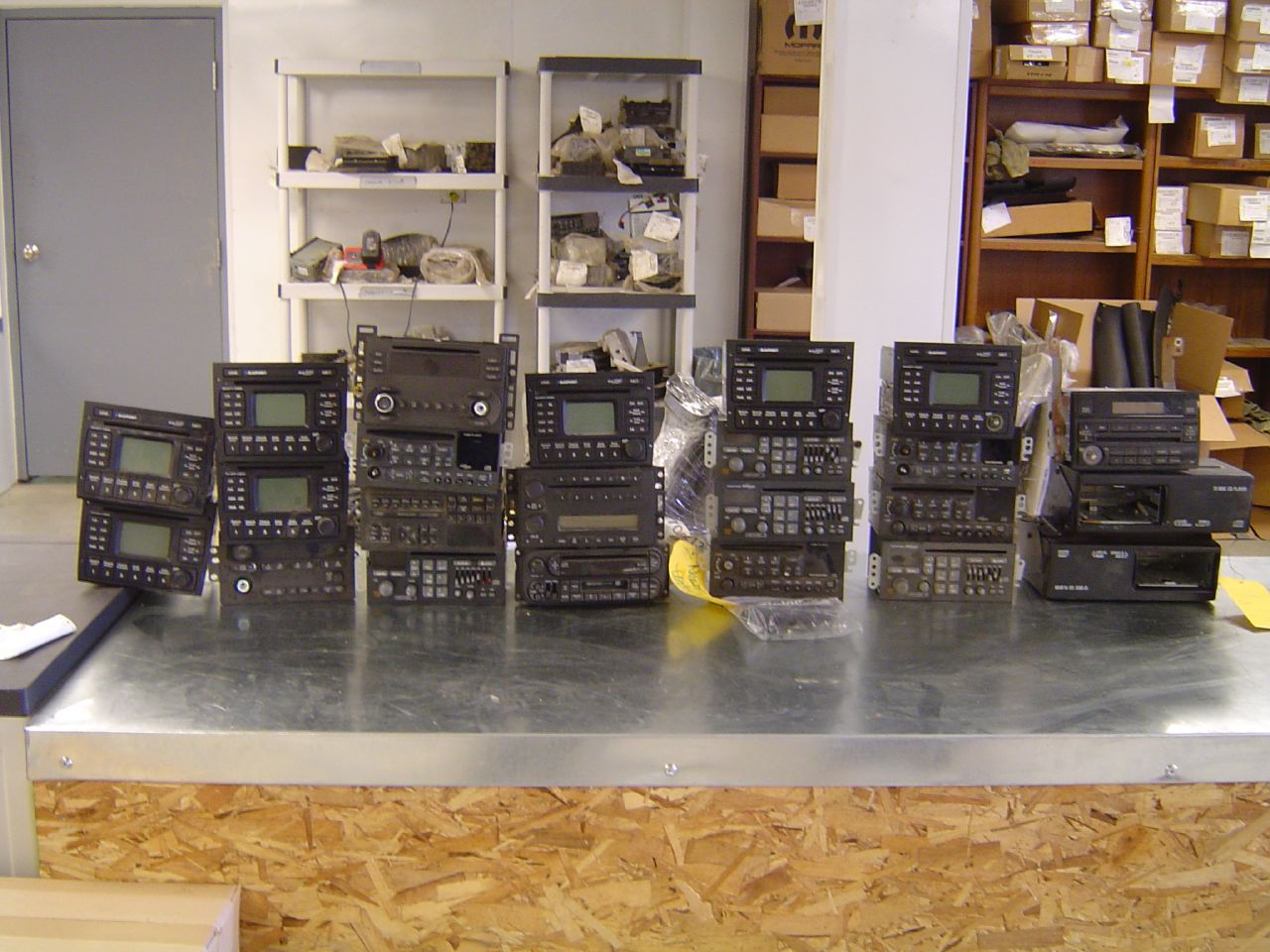This color photograph captures a cluttered storage room with a stainless steel countertop that has a particle board front. On the countertop, there are seven stacks of black car stereos, each stack varying between two and four units high. Each stereo features digital displays, buttons, and some knobs, mostly in black. In the background, to the left, a gray door with a silver knob is visible. Adjacent to the door, there are white plastic shelves laden with various unidentifiable items. Further to the right, brown wooden shelves are packed with brown boxes, many adorned with invoices or shipping labels. A white support post is also visible amidst the shelving units.